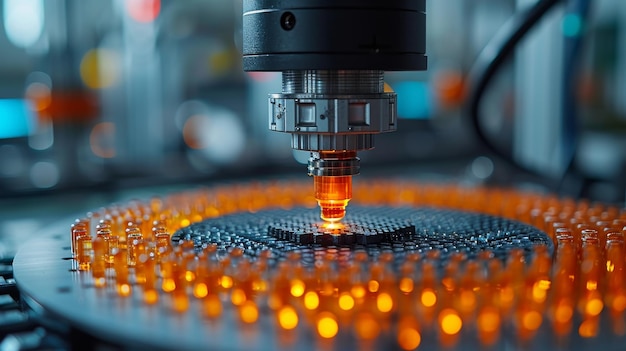The image depicts a highly detailed mechanical apparatus, likely a modern laser stamping machine, operating within an industrial setting. Central to the composition is a tubular black object extending from the top, about an eighth of the way down into the picture plane. Attached to this central cylinder is a series of silver components that taper into a smaller structure with a prominent orange tip, suggesting it may be a laser emitter. This apparatus is in sharp focus, in contrast to the background which is thoroughly blurred.

The orange-tipped device appears to interact with a multi-layered black pad, which is slightly raised and textured. This pad transitions into another black surface, dotted with several amber-colored pins that resemble illuminated inserts or possibly Light Brite pegs. These pins are arranged within a circular metal plate punctured with holes, adding complexity to the machinery.

Illumination seems to come from behind the machine, casting some light towards the front but leaving many details indistinct. The overall lighting accentuates the metal and plastic components, contributing to the photorealistic representation of the device. While the exact function remains ambiguous, the emphasis on the laser tip and surrounding elements suggests a high-precision task, possibly engraving or intricate cutting, taking place in a workshop environment.